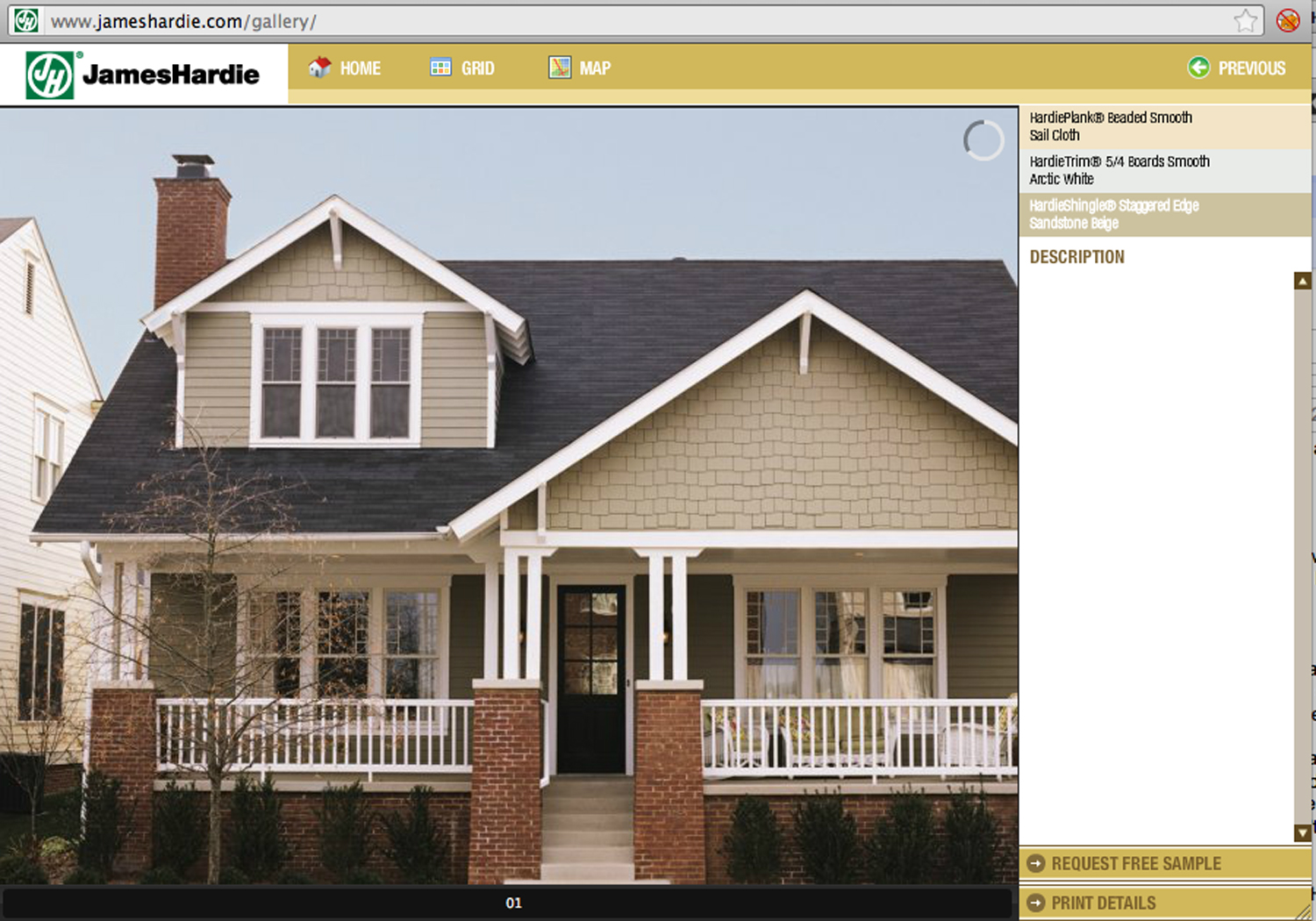The screenshot shows a webpage from the URL www.jameshardie.com/gallery, displaying an image of an American-style house. At the top of the screen is a green icon in a square with a white circle and letters “JH,” indicating the website, with navigation options labelled "Home," "Grid," and "Map" beside icons. A back button with a green circle and white arrow, along with the word “Previous,” is found on the upper right. The right side of the screen is partially covered by a text strip and a scroll bar, with additional golden buttons in the bottom right corner.

The main image showcases a large, multi-level house with various architectural details. The house features a dark, pitched roof with grey shingles and a brown brick chimney on the top left. The attic area includes a dormer window with three vertical panes, framed in white. Below, there is a prominent front porch with white fencing about a foot high and a black door with a six-pane glass arrangement in a two-by-three vertical grid. Brick columns flank the porch's sides, supporting white columns above. The house's exterior includes sections of beige-brown paneling and white trimming around the windows. In front of the house, small dark hedges line the brick base, and a barren tree stands to the left. Part of a neighboring house with white paneling is visible on the left side of the image. The property also features large windows and balcony areas, with small trees lining the front path.